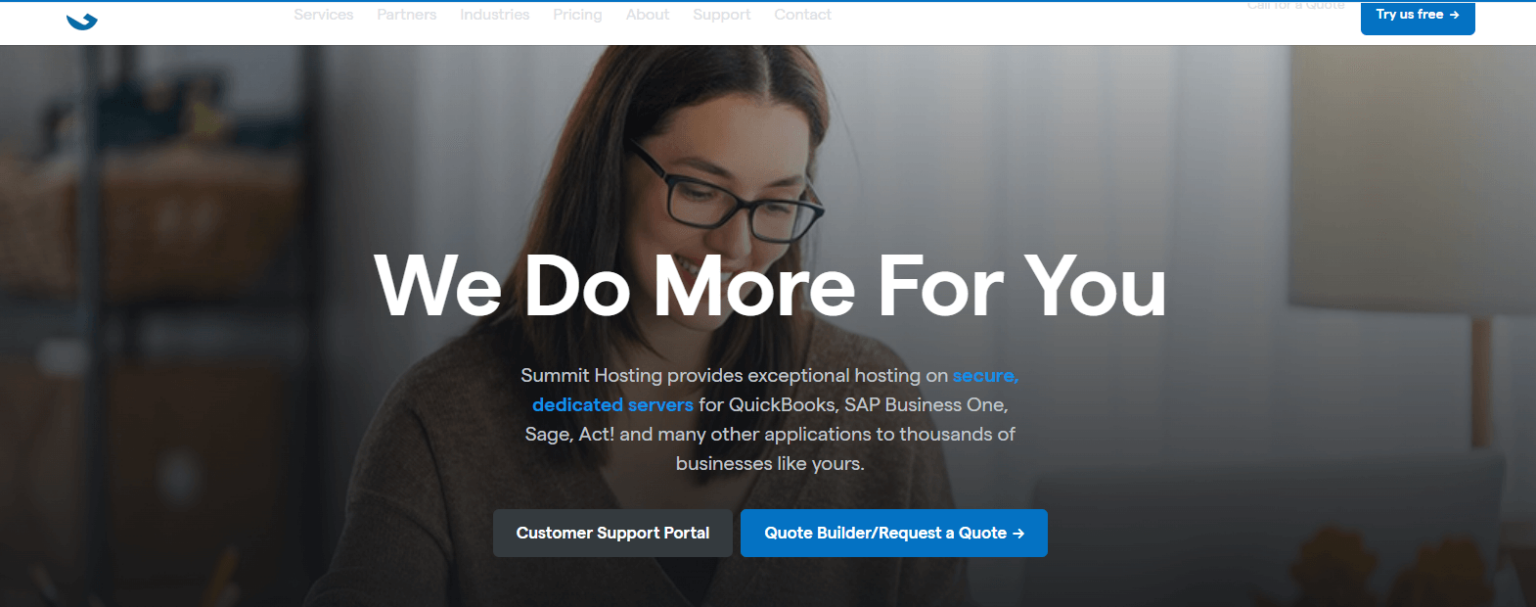The image is a screenshot of a website. At the top of the screen, there is a horizontal blue line. Below this line, the background is white with a small blue logo resembling a crescent moon. In the upper right corner, there is a button labeled "Try Us Free." To the left of this button, in light gray text, are the following menu options: "Services," "Partners," "Industries," "Pricing," "About," "Support," and "Contact."

The main section of the screenshot features a color photograph of a young woman with long brown hair. The photo shows her from the chest up; she is looking down, smiling, and wearing a pair of glasses and a blazer. Overlaying the image, in large white block-style text, are the words "We Do More For You."

Beneath this, in smaller gray text, is an informative description: "Summit Hosting provides exceptional hosting on secure, dedicated servers for QuickBooks, SAP Business One, Sage, Act, and many other applications to thousands of businesses like yours."